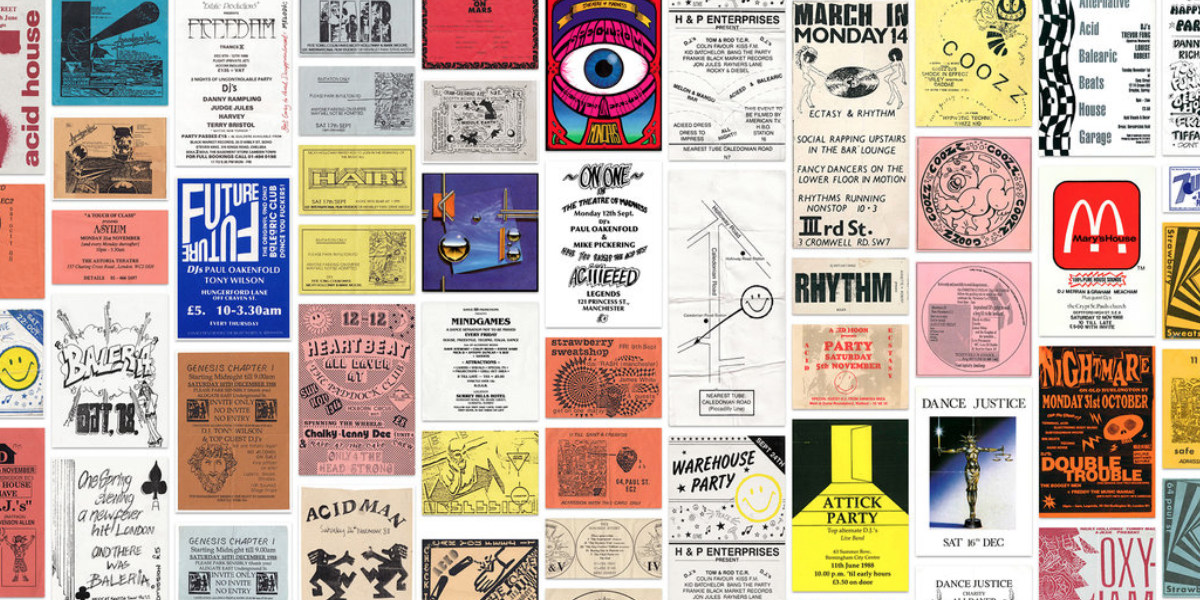The image is a vibrant collage consisting of numerous small, rectangular images arranged closely together, resembling a poster or placemat filled with various ads and colorful graphics. Predominantly set on a white background, the collage features a diverse color palette including shades of blue, pink, purple, tan, black, cream, and red. 

Among the numerous images, one prominently features the words "acid house" in red letters on a white background. Another highlights the word "future" on a blue background with white lettering. A distinct image showcases the phrase "acid man" on a cream-colored background with black text, and another contains what appears to be test tubes set against a purple backdrop. There are additional elements within this eclectic mix, such as an eyeball, a smiley face, and representations of people, including one holding a record disc, a statue resembling a trophy, a skull, and a baby.

Vertically-oriented text and ads are apparent, such as "ballerina" appearing in one section, "freedom," "future," and event advertisements like "October 18th." There are also references to party and music cultures with phrases like "attack party," "warehouse party," "nightmare," and "double trouble." Familiar brand imagery is present, including an ad for McDonald's. Overall, the arrangement of these images creates a dynamic and visually engaging collage that showcases a variety of artistic styles and textual elements.